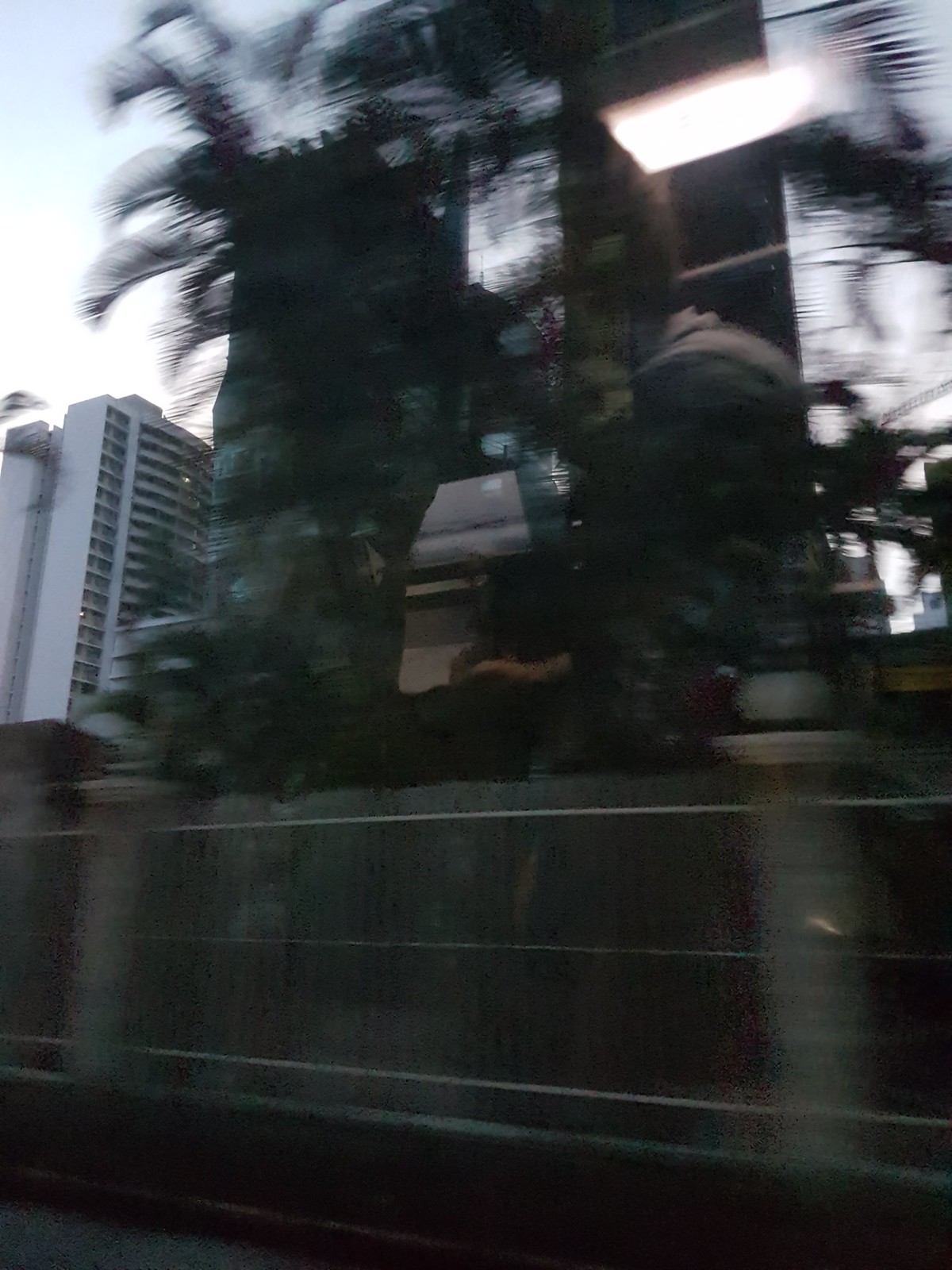The image showcases a dynamic scene likely captured from inside a moving vehicle, potentially a bus, evident from the slight motion blur. Central to the image is a reflective glass display, which mirrors parts of the background. On the left, a towering building with a park-like structure is visible, featuring multiple rooms and balconies. The sky above is predominantly blue with scattered white clouds, extending to the far right side of the image. In the foreground, lush green plants are seen near the base, interspersed with a fence made of stone pillars connected by metal grates. The overall setting gives a sense of urban vibrancy contrasted with natural elements.